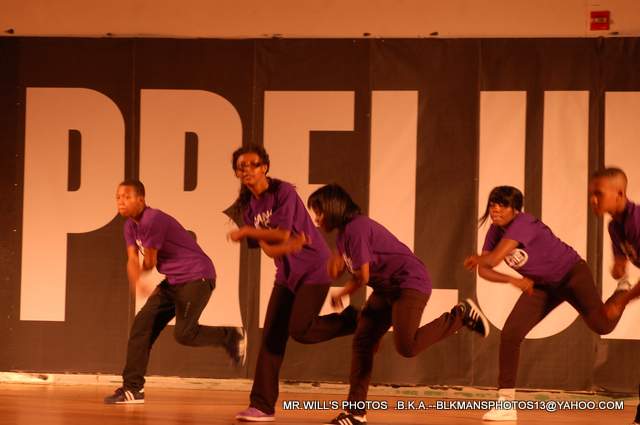The photograph showcases a dynamic dance scene featuring five high school students—four teenagers and an older individual, all part of an African-American dance troupe. They are arranged on a wooden stage, each dressed in purple t-shirts, dark jeans, and sneakers. Their energetic pose captures them balancing on one foot, arms in motion as if performing a barrel roll, mid-dance. The backdrop features large, partially obscured letters spelling out "PRELU," likely part of the word "prelude." Overhead, warm yellow lighting, typical of gymnasiums, illuminates the scene. In the bottom right corner, a watermark reads: "Mr. Will's Photos, BKA, BLK, mansphotos13 at yahoo.com."